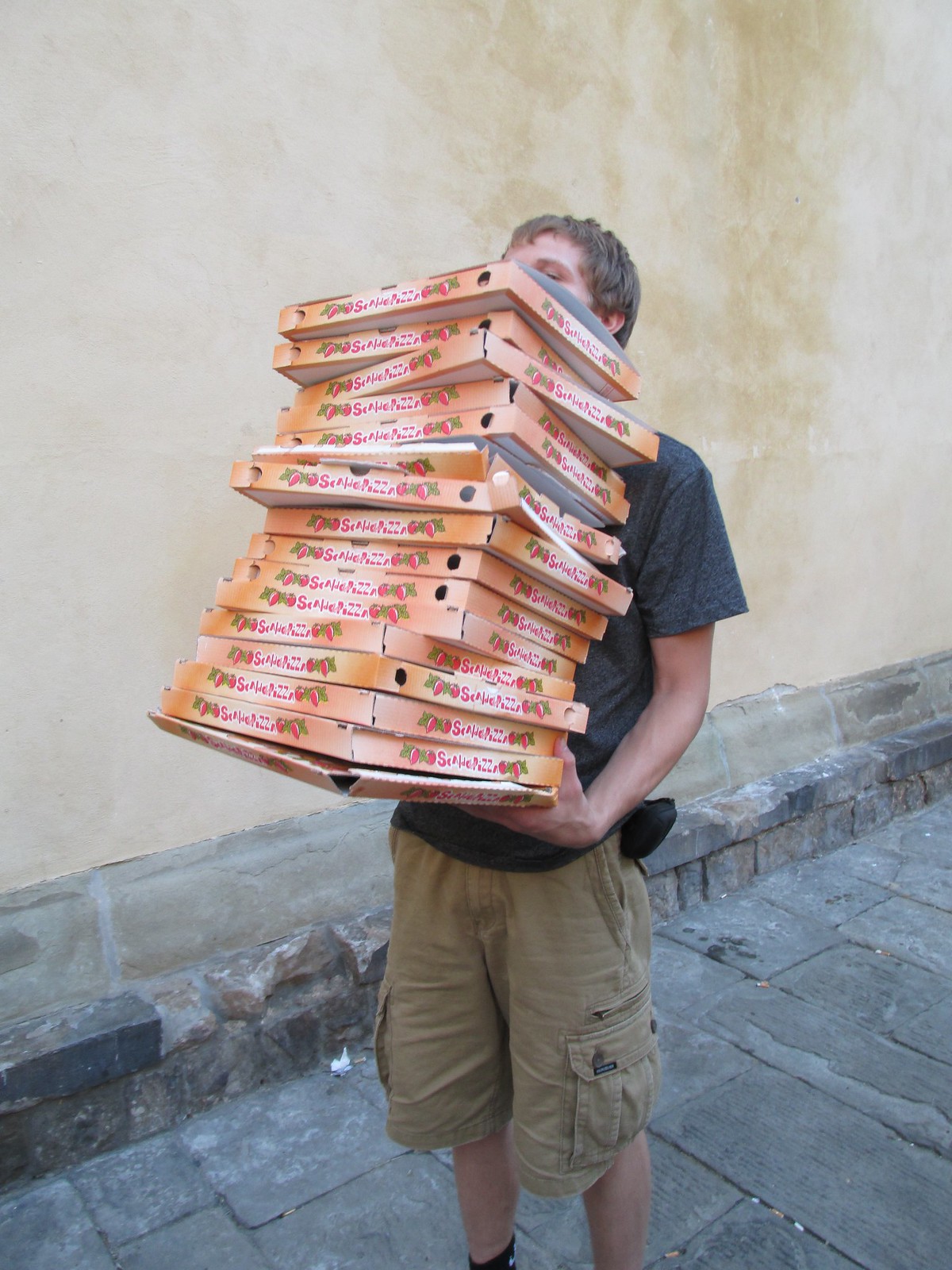In this photograph, a young Caucasian man with short light brown hair is standing outside near a beige plastered wall that has a stone lining at the bottom. He is dressed in khaki cargo shorts that extend beyond his knees, a gray short-sleeved t-shirt, black socks, and partially visible shoes. A pouch, possibly a fanny pack, hangs off the rear left side of his shorts. His arms are outstretched in front of him, holding a towering stack of pizza boxes — approximately 15-20 in total, which obscure most of his face, revealing only his left ear and eye. The pizza boxes are flesh-toned with red hand-written type flanked by illustrations of tomatoes or peppers. The setting suggests he is either delivering or transporting these pizzas along a paved street adjacent to the wall, where he has momentarily paused for the picture.